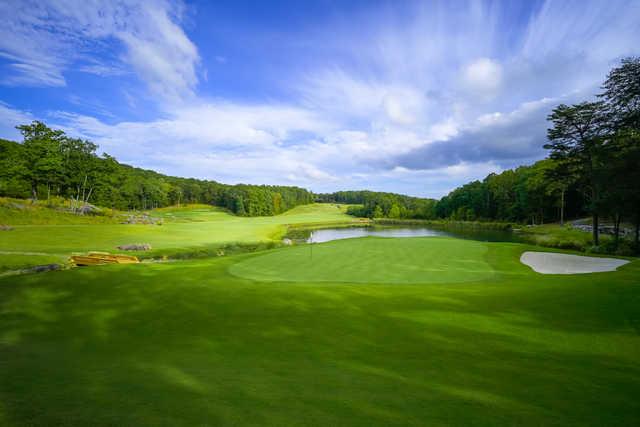The photograph captures a serene and picturesque golf course under a partly cloudy, blue sky. In the foreground, a lush, perfectly maintained green with a flagstick marks one of the holes, accompanied by a sand trap to the right. A small wooden bridge spans a water hazard, dividing this hole from another visible fairway, which features slightly lighter green grass. Surrounding the course, a dense line of forest trees adds to the natural beauty. The calm pond and orderly fairways exhibit the course's meticulous upkeep, while the overall scene radiates tranquility with no golfers in sight, allowing the pristine nature of the course to stand out.